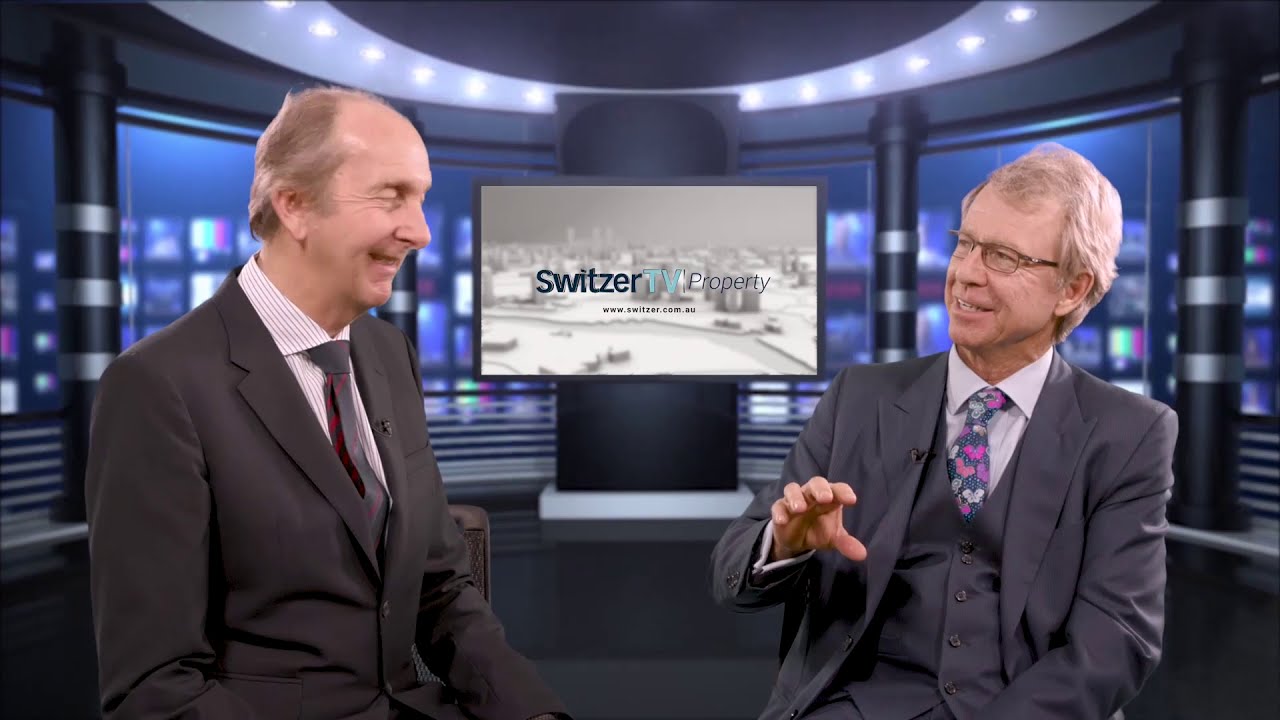In this detailed image from a TV or news studio with a curved, black-and-blue themed backdrop, two older white males are engaging in a lively conversation, filled with laughter. The man on the left is dressed in a dark gray suit with a white, black pinstriped button-down shirt and wears a black tie featuring a subtle red pattern. He is balding with gray hair at the back of his head. The man on the right, sporting rectangular black eyeglasses, is wearing a light gray suit with a matching vest, complemented by a white button-down shirt and a multicolored tie adorned with Mickey Mouse ears. The studio background features a prominent black pillar with a mounted large TV screen displaying the words "Switzer TV Property," set against blue screens and black poles that add to the high-tech ambiance.